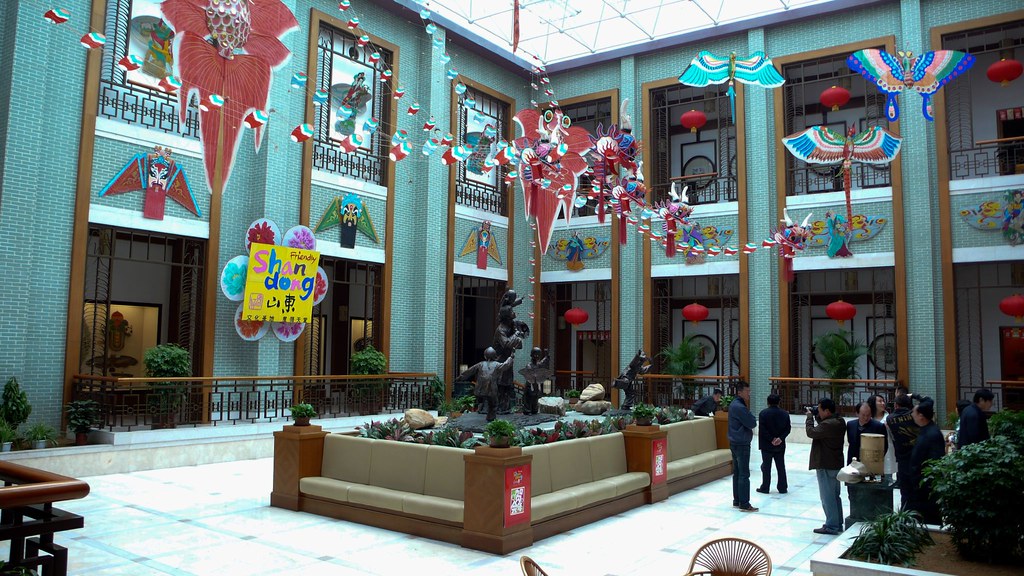In the image, an indoor kite museum features a quadrangle design with a transparent glass ceiling, allowing natural light to flood the space. The museum comprises two green buildings, joined together at a right angle, adorned with a variety of kites and intricate wall designs. In the foreground on the bottom right, a group of tourists, identifiable by their cameras and tour guide, are taking photos. Central to the quadrangle is a rectangular fountain surrounded by tan sofas for seating. The fountain features bronze statues of children reaching up. The ground is paved with blue tiles, and the space showcases several artistic elements including kimono displays with kabuki masks, phoenixes hanging from the ceiling, and strings decorated with red and teal eggs. The left part of the building bears a yellow square banner with the words "San Dong."